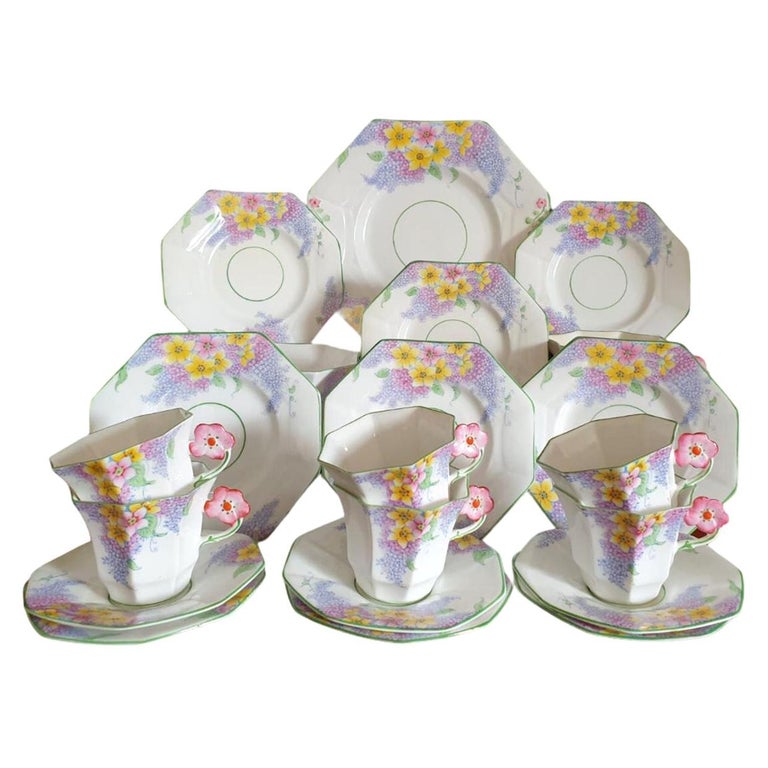The image displays a partial set of elegantly detailed china teaware, featuring an octagonal shape across all items, including plates, saucers, and teacups. The backdrop is a simple white, likely intended for catalog or listing purposes. This set includes one large serving platter at the back, followed by three progressively smaller dinner plates, and a row of three salad plates. Additionally, there are two sets of two teacups stacked on saucers placed at the front. 

Each piece in the set is predominantly white with a green circle in the center and green edging. The design features a floral pattern, dominated by five-petal yellow flowers surrounded by various smaller blossoms in shades of pink, purple, and blue, along with green leaves. Notably, the teacups have a unique handle adorned with a ceramic pink flower with a red center, ergonomically placed where the thumb rests. This intricate and cohesive floral motif, combined with the pastel color palette, exudes a vintage charm reminiscent of dishware styles from the 1960s to the 1980s.